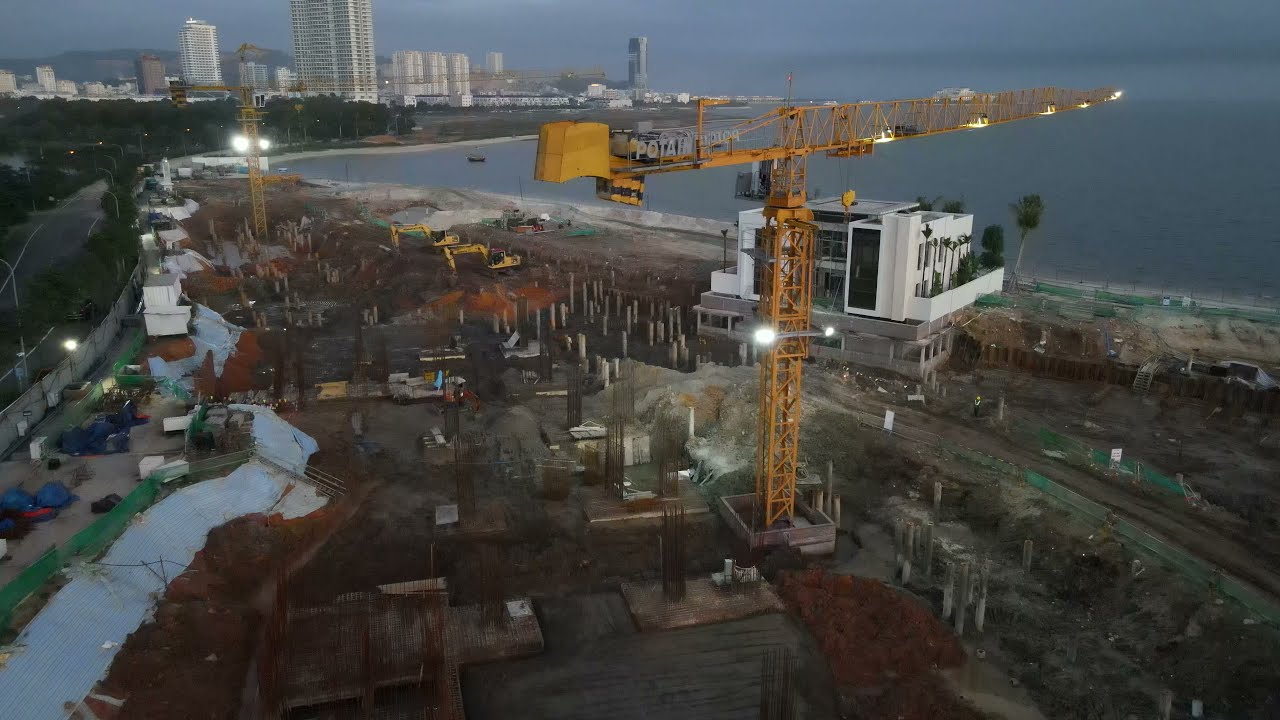High above a bustling construction site, the overhead view captures a vivid scene dominated by a large, orange-yellow crane, angled at about the 1:30 to 2 o'clock position. The crane stands out prominently, with its detailed structure showing a white and gray platform. The ground below is a freshly moved expanse of brown dirt, sparsely populated with pillars and other construction equipment, including several backhoes. The left side of the image reveals an undeveloped area lined with trees, while the far background displays a cityscape featuring skyscrapers and commercial buildings. This urban sprawl extends towards a peninsula jutting into a vast body of water, possibly an ocean, in the upper right. The sky above is a medium blue, nearly blending with the water below, creating a tranquil backdrop to the industrious activity below.